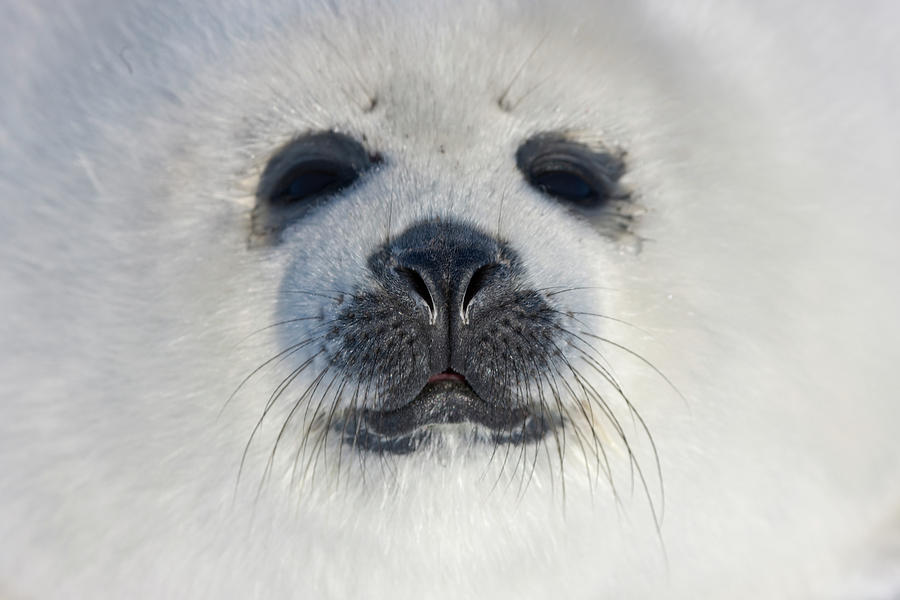This is a close-up photograph of a seal pup's face, which occupies the entire horizontal rectangle frame. The pup has strikingly pure white fur that extends outward in many fine strands, making the animal appear almost entirely white. Its big, glossy black eyes are rimmed with darker shades and a few delicate white lashes. The seal’s black nose features small, slanted nostrils, and black whiskers fan out from the base of its nose, hanging down alongside a small, somewhat pursed black mouth, from which a tiny glimpse of its pink tongue is visible. Some subtle detailing includes a slight shadow on its forehead and some dark shading surrounding its eyes and mouth. The background and body of the seal are blurred, ensuring all focus remains on the detailed and well-lit facial features, suggesting the photo was taken during the daylight, possibly in an icy, cold environment like Antarctica.